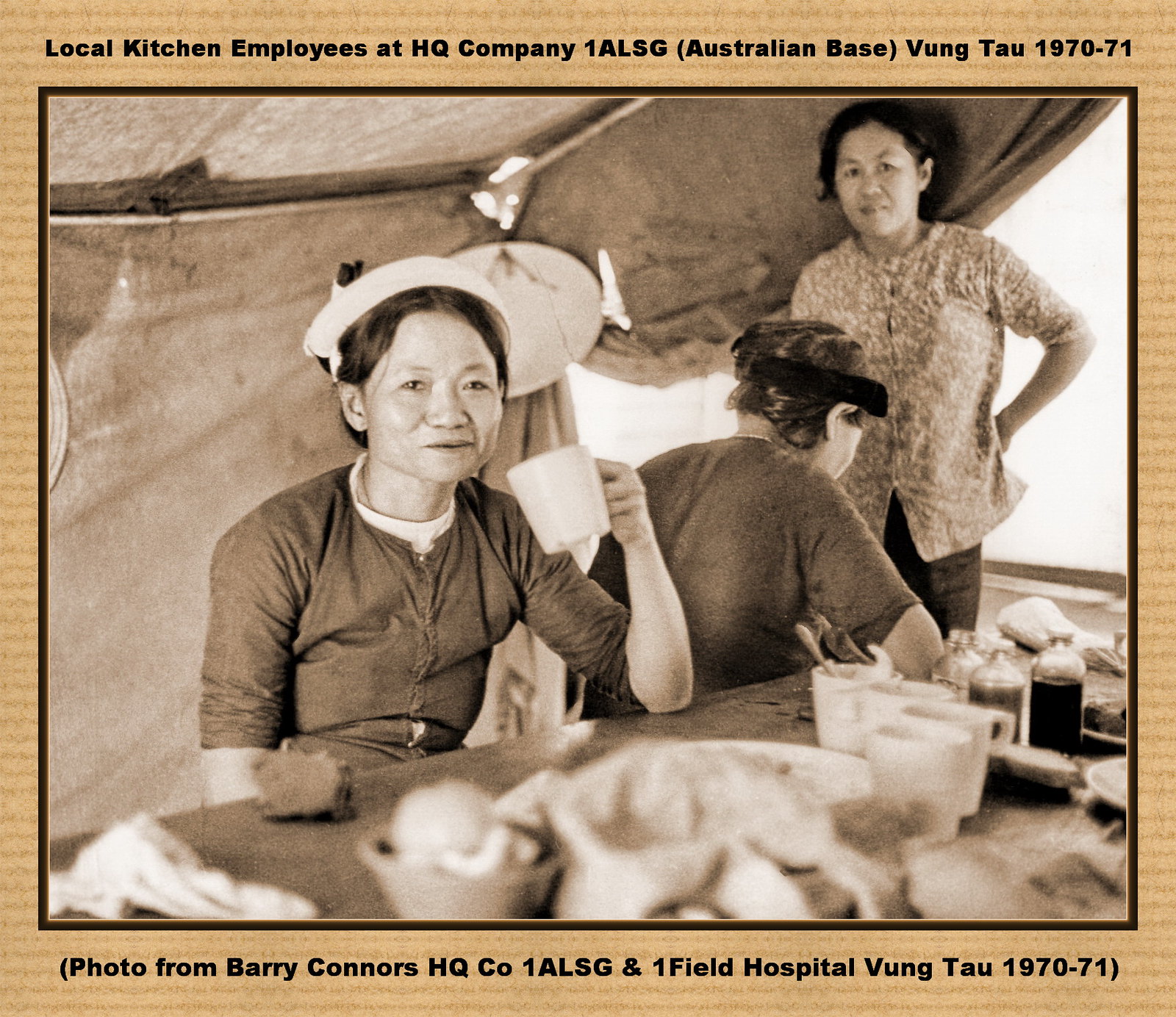The image is a black-and-white photograph from 1970-71, showcasing three elderly Asian women inside a tent at the HQ Company 1ALSG Australian base in Vung Tau. The tent has an open front and covered sides and top, creating a makeshift indoor setting. The photograph, surrounded by a tan corrugated border, features a headline and caption indicating its historical context, "Local Kitchen Employees at HQ Company 1ALSG Australian Base Vung Tau 1970-71" and "Photo from Barry Connors, HQ CO 1ALSG and 1 Field Hospital Vung Tau 1970-71."

One woman sits at the forefront, resting her elbow on a wooden table filled with various dishes, including three cups—one with a spoon—and three bottles filled with liquid. She wears a light-colored hat or visor and a solid cardigan while holding and drinking from a white mug, smiling at the camera. Another woman, seen from behind, sits next to her, donning a floral cardigan and a nurse’s cap. A third woman, also wearing a nurse’s cap and dark gray sweater, stands in the back, looking at the viewer. The vintage landscape photograph, capturing a candid moment of camaraderie, reflects the everyday lives of kitchen employees during that era.